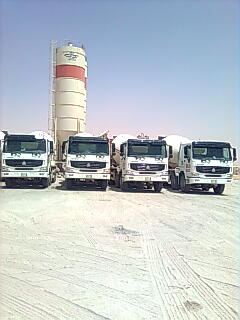The photograph captures a lineup of four large white trucks, facing directly towards the photographer, their black grilles set against sizable front windshields that stretch entirely across the cab. The trucks appear cube-like, with one truck on the far right slightly angled, revealing a prominent front wheel. Each truck has a cylindrical drum on its back, suggesting they might be cement mixers or possibly used for gas or liquid storage. The vehicles are parked on a ground that looks like white sand or dirt, marked with numerous tire tracks, indicating a well-used area. Above, the sky transitions from a clear blue to a hazy pink near the horizon, suggesting it's likely taken around mid-day due to the brightness. In the background, a tall, thin white tower with a ladder along its left side and a distinctive red stripe running across its upper section stands against the sky, contributing to the industrial atmosphere of the scene.